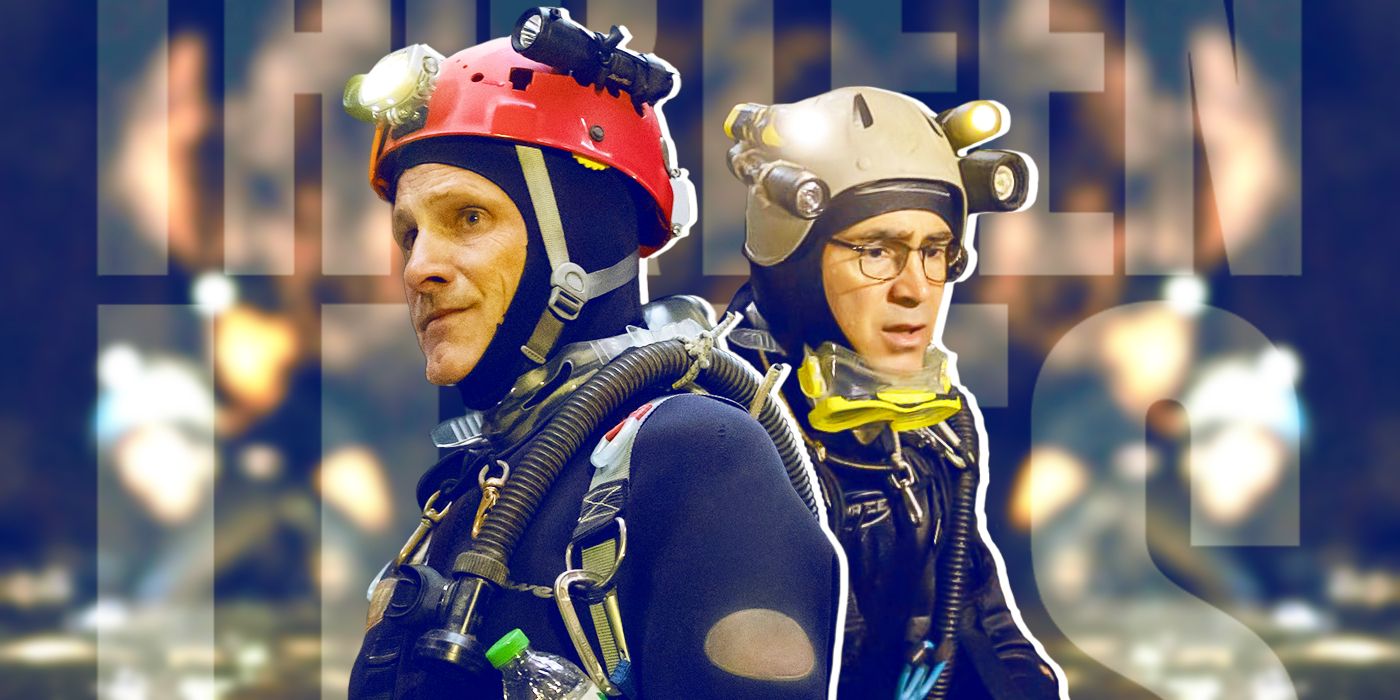This detailed descriptive caption combines the information provided from both voice descriptions, emphasizing the shared elements:

The image depicts a promotional movie poster featuring two men in scuba gear, both adorned with helmets equipped with flashlights. The man in the foreground, on the left, wears a red helmet commonly used by rock climbers, featuring a black flashlight attached to the side and a headlamp at the front. He is joined by another man partially visible behind him, who dons a tan-colored helmet, adorned with two side-mounted flashlights, and yellow goggles draped around his neck. This man also wears eyeglasses and a black scuba suit. Dominating the background is large, projected text that appears to spell out '13 Lies,' reflecting the title of the movie and creating a light effect on the wall. The overall ensemble of the gear and the dramatic lighting, alongside the obstructed text, underscores the promotional nature of the image, highlighting its purpose as an advertisement for the film.